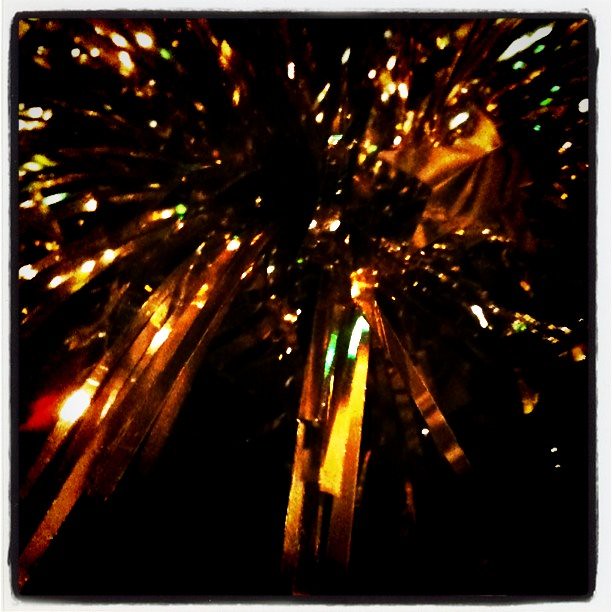The image features a strikingly artistic display set against a very black background. At its core, it resembles a cheerleader's pom-pom, with numerous reflective surfaces that radiate outwards from the center. The materials appear to be highly reflective, possibly metallic or cellophane, capturing and dispersing light into a mesmerizing radial pattern. The central elements gleam with a spectrum of colors, predominantly brownish gold, with accents of yellow, pink, orange, and hints of green and blue. The light bounces off these surfaces, creating sharp dots and speckled reflections that seem to float in a vortex-like formation. The interplay of light and material forms an intricate display, with the central area remaining dark, enhancing the contrast and depth of the scene. The entire composition is enveloped in darkness, drawing attention to the luminous, colorful display at its heart.